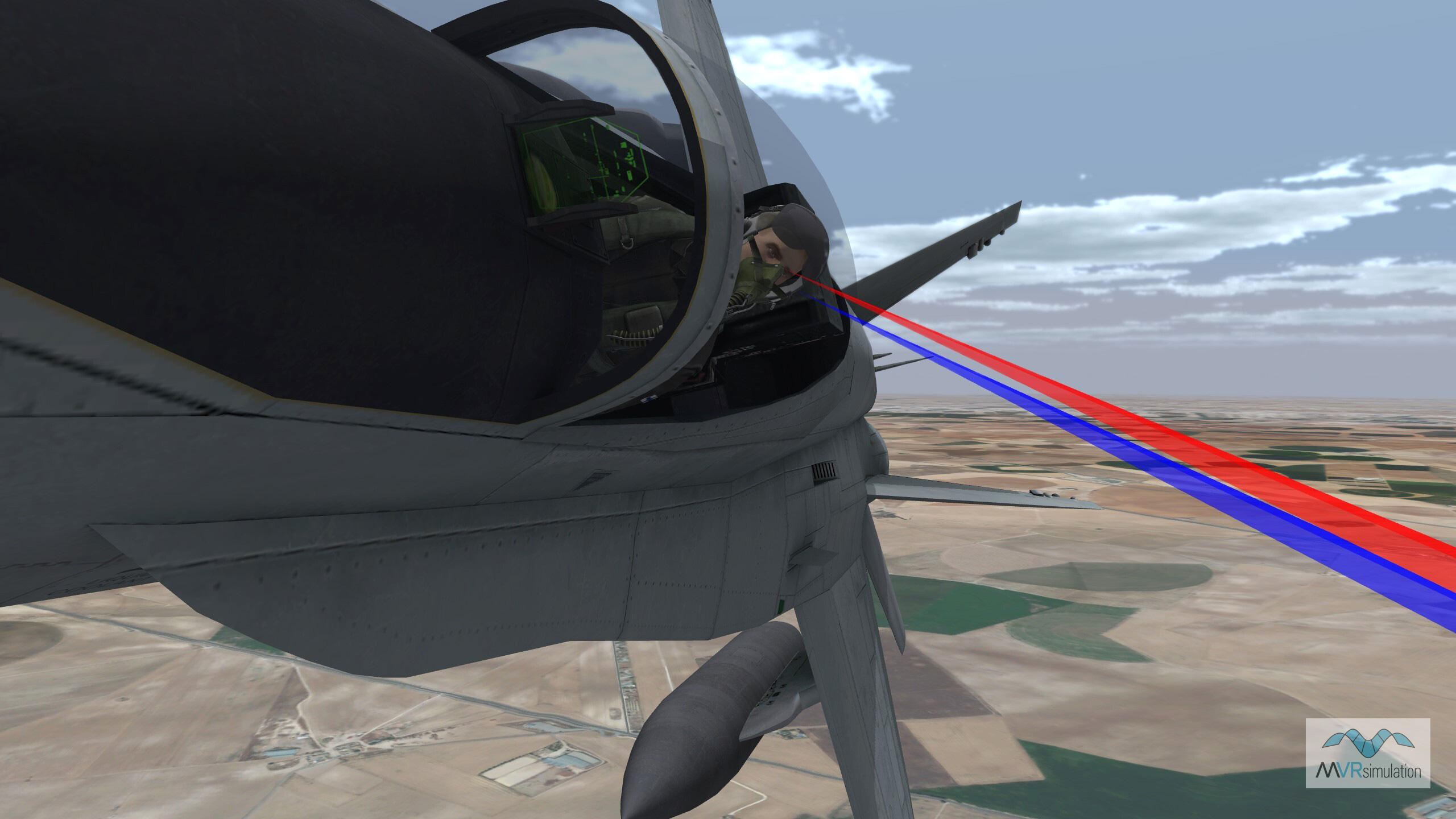This is an image from the game Microsoft Flight Simulator showing the cockpit of a small, gray airplane in flight. The scene is viewed from the pilot's perspective, who is dressed in a flight suit and appears to have black hair. The cockpit's instruments, including green dials, are visible, but the area is heavily shadowed, rendering most of it nearly black. The pilot is gazing intently to his left and downward, where there are two colored lines - one red and one blue - seemingly emanating from his eyes. These lines extend toward the center of the image, possibly indicating a focus area or a simulated target.

The landscape below is a geometric patchwork of tan land with green squares and lighter green designs, intersected by gray lines that resemble roads. The horizon transitions into a light gray sky with streaky white clouds that gradually become a blue-gray color. The plane appears to be at a considerable altitude, possibly during takeoff or landing, as the ground patterns and what looks like a runway are visible below. The image is low-resolution, adding a somewhat pixelated texture to the visual elements.